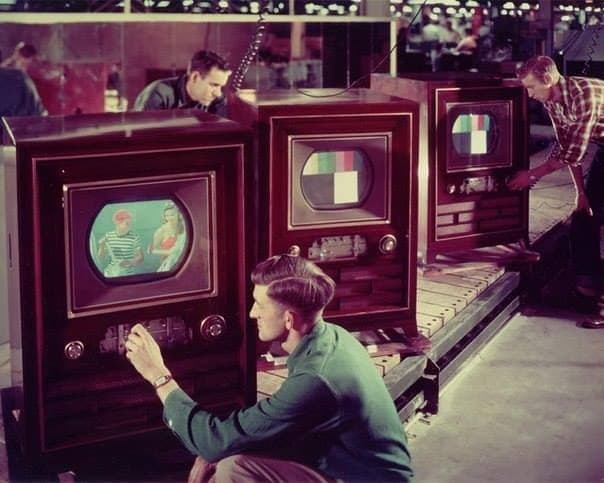In this image, we see a 1950s TV store or possibly an assembly line, showcasing three old-style televisions encased in ornate mahogany-colored wooden boxes. Each television features a small, curved screen on the sides and flat on the top, surrounded by buttons and knobs for tuning and adjustment. The screens display colored pictures, with the left-most TV showing an image of a red-haired boy in a striped shirt talking to a brunette lady in a red sleeveless dress.

In the foreground, three Caucasian men are interacting with the TVs. The man on the left, wearing a blue shirt with a wristwatch, is squatting down and adjusting the panel with his left hand. The man on the right, dressed in a plaid shirt, is standing and touching the dial of the right-most TV. A third man, wearing a dark shirt, is seen behind the middle TV, squatting and looking at it intently. The setting appears to be an old showroom or factory, with the TVs placed on a low wooden platform, suggesting they are either being tested or displayed for customers.